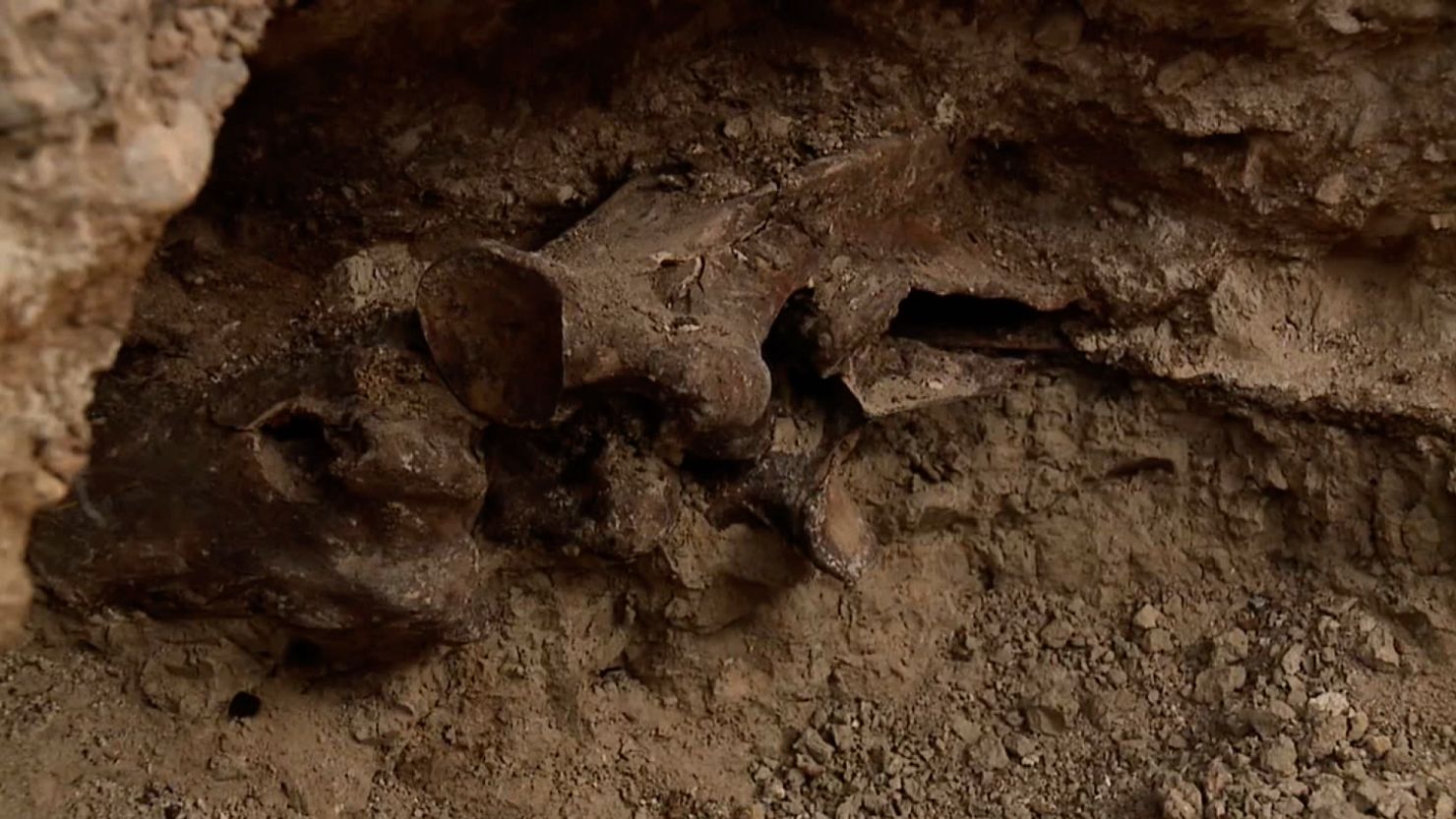The photograph captures a close-up scene inside a cave, featuring an archaeological dig site dominated by varying shades of brown, taupe, and gray. The foreground reveals crumbled dirt and various rocks, while darker cavernous nooks create a sense of depth. Central to the image is a partially unearthed artifact, resembling a metal pitcher, with its opening just visible amid the dirt and sediment. Adjacent to it, another piece of material, possibly metal or wood, is also discernible, suggesting it is part of the same find. Additionally, there are elements peeking out of the dirt that could be bone or rust, including what appears to be a small skull partially covered by the earth. The scene is rich with textures and layers, indicative of an ongoing excavation process with much of the discoveries still embedded in the surrounding mud and clay.